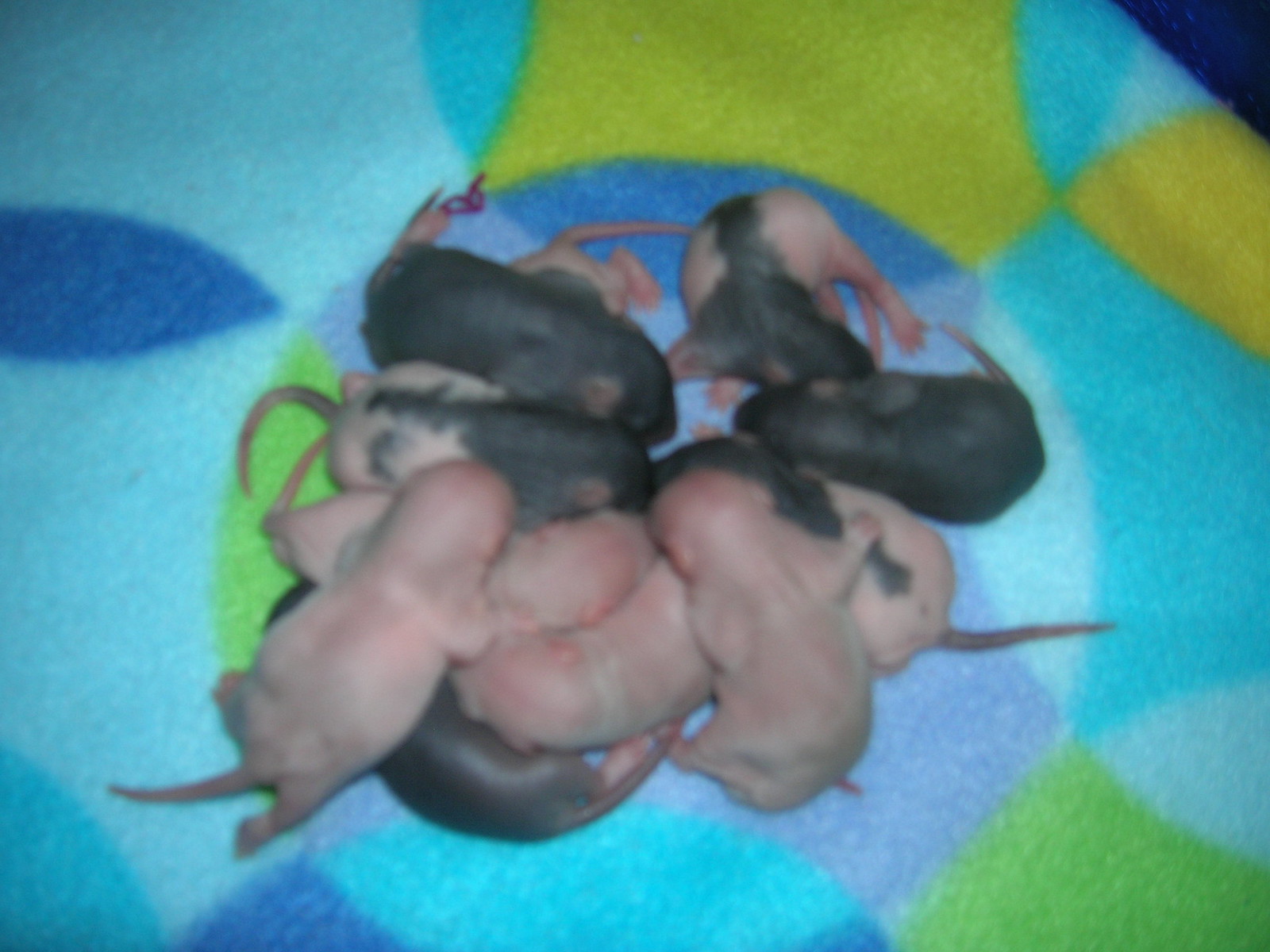The photograph features approximately 12 newborn baby animals, potentially mice or rats, nestled closely together in a communal sleep. Their delicate, hairless bodies exhibit varying colors, with some being tannish pink, others black, and a few showcasing a combination of pink and black hues. These tiny creatures have long, pink tails and visible little pink ears, along with arms and legs. They are all lying atop a soft, multicolored blanket with geometric patterns in blue, yellow, green, and possibly purplish and teal tones. The babies are adorably snuggling and holding onto each other, creating a heartwarming scene of togetherness and innocence. The background is free of text, and the exact nature or timing of the image remains unspecified.